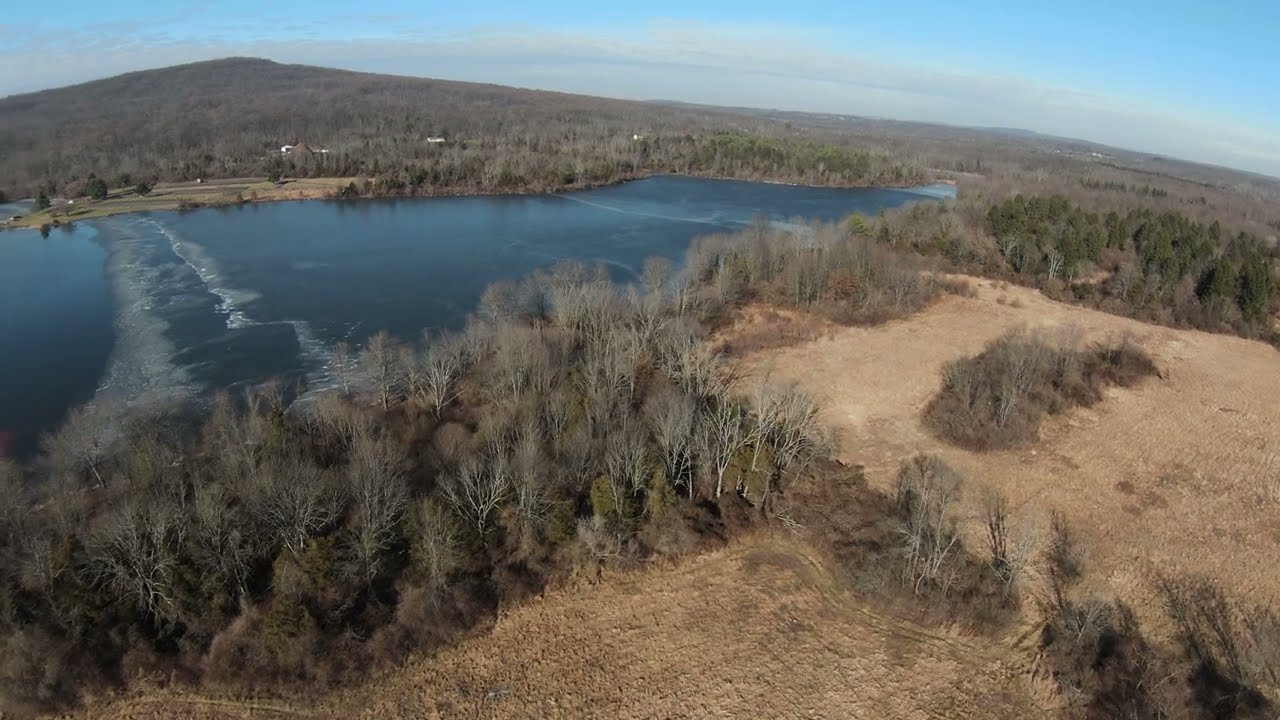In this high-angle, elevated shot—likely taken from a drone—there's a vivid and expansive winter landscape below. The central focus is a large, partially frozen blue lake, around which the geometric patterns of ice cracks are clearly visible. Surrounding the lake, there’s a combination of bare trees and scattered evergreens, indicative of the winter season with most foliage absent. On one side of the lake, stretch expanses of plowed farmland, marked by freshly turned brown soil, devoid of crops. Adjacent to the farmland and closer to the lake’s edge, a small forested area acts as a natural boundary. As the scene extends outward, denser forested areas and some residential zones become visible on the opposite shoreline. The sky above is a crisp blue, interspersed with clouds, further emphasizing the chill of the season. The overall scene captures a serene yet stark natural beauty, blending the earthy tones of bare soil and leafless trees with the icy tranquility of the frozen lake.